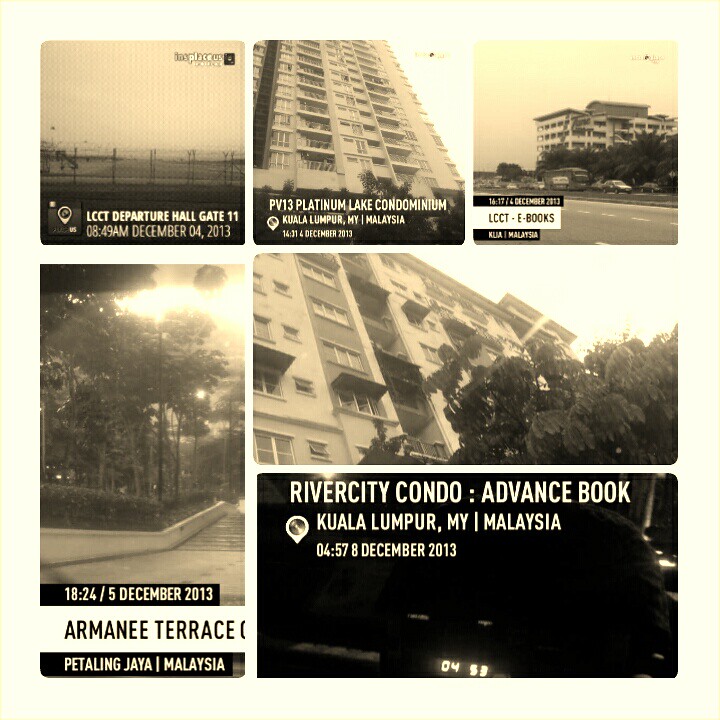The image is a large square collage with a beige background and a faint tan border, featuring six black-and-white and sepia photographs arranged in two rows. The top row consists of three square images: the left one shows a fence and sky with the caption "LCCT Departure Hall, Gate 11, 8:49 a.m. December 4th, 2013"; the middle one depicts a tall building labeled "PV13 Platinum Lake Condominium, Kuala Lumpur, MY/Malaysia, December 2013"; the right one illustrates a street with a complex building and states "LCCT eBooks, December 2013, Malaysia." The bottom row contains three rectangular images: the left vertical rectangle shows a walkway with trees labeled "5 December 2013, Aramani Terrace, Petaling Jaya/Malaysia"; the middle horizontal rectangle presents part of a tall building with trees in the foreground, without text; and the right horizontal rectangle, darker than the others, displays illuminated numbers "453" and reads "River City Condo Advanced Book, Kuala Lumpur, MY/Malaysia, 4:57, 8 December 2013."